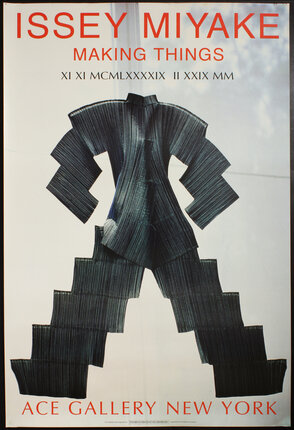This advertisement shows an image against a whitish-gray, cream-green background with a cloudy sky impression. Dominating the top, bold red text spells "ISSEY MIYAKE" with "making things" beneath in smaller red letters. Following that, in smaller black text, it reads "XIXI MCMLXXXIX MM." Below this text, in the center, there's a striking design resembling a human figure crafted from rectangular sections. The figure, appearing in dark gray tones with lighter striated lines, wears what looks like a suit, missing a head. The upper part resembles a shirt or coat made of rectangular shapes, while the lower part features pant legs in an upward step-like accordion fold pattern. Surrounding this image is a black border framing the setup. Finally, at the bottom, "Ace Gallery, New York" is written in red text, anchoring the ad.